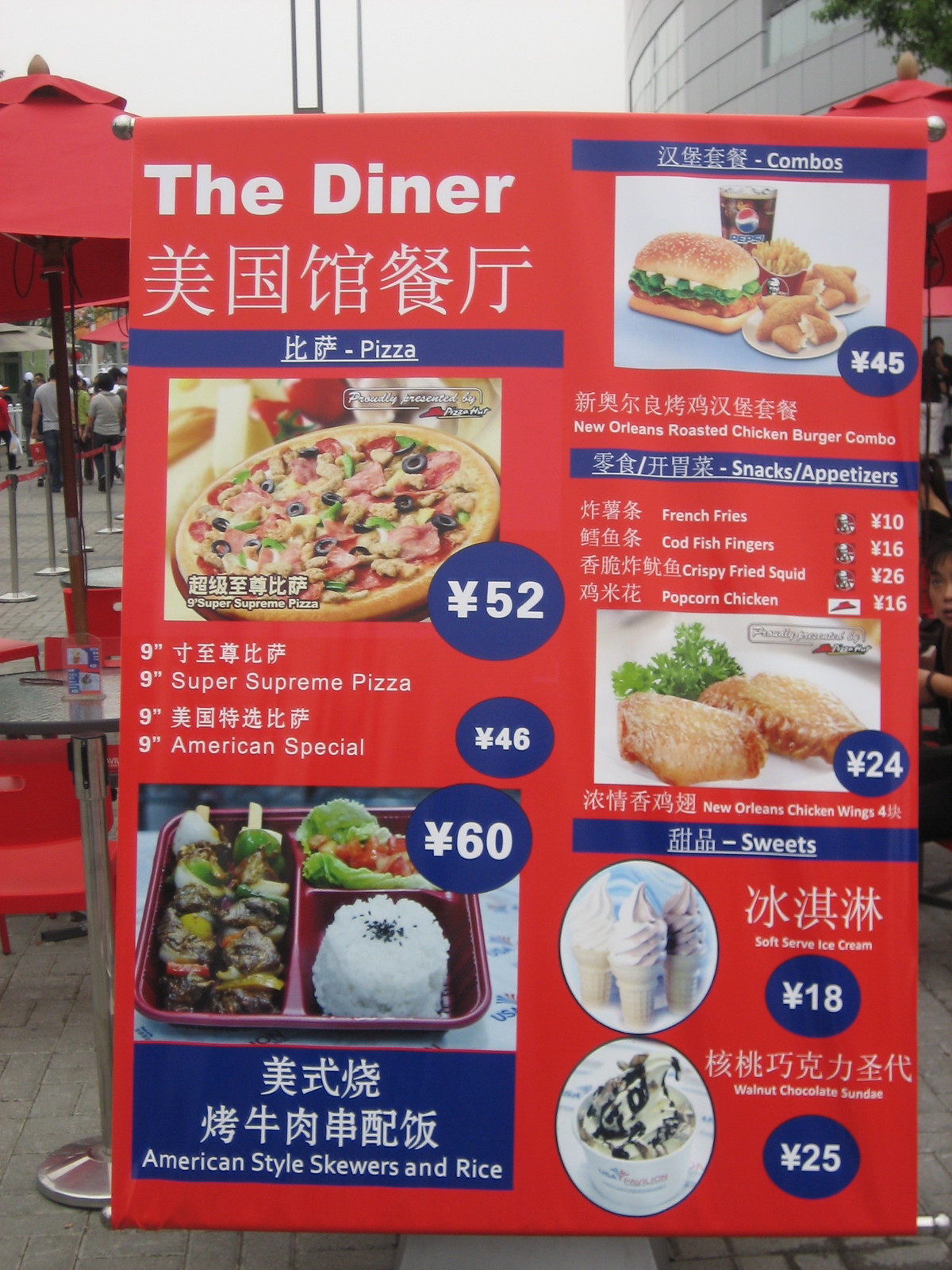In the bustling streets, a large rectangular diner poster being mounted on sturdy aluminum poles captures attention with its vibrant design. The poster predominantly features a rich red background, punctuated at the top with the diner's name displayed prominently in white lettering, accompanied by Japanese writing beneath it. 

A striking blue band runs horizontally, showcasing a mouth-watering image of a pizza. Adjacent to the picture, the price is clearly indicated in white numbers within a blue circle – 52 yen. The poster meticulously lists various nine-inch pizza options, including a "Super Supreme Pizza" and an "American Special," both priced at 46 yen, highlighted in a similar blue circle.

Further down, the poster tantalizes with a photograph of an American-style skewer served with rice, again set on a blue section. Above this image, the price is noted as 60 yen within a blue circle. A section for combo deals follows, priced at 45 yen, featuring appetizing visuals of snacks and appetizers available for 24 yen.

The bottom of the poster sweetly concludes with a variety of dessert options. Soft serve ice cream is attractively priced at 18 yen, while a walnut chocolate sundae is offered for 25 yen. The detailed imagery and clear pricing on the poster make it an inviting beacon for hungry passersby, promising a range of delicious and affordable delights.